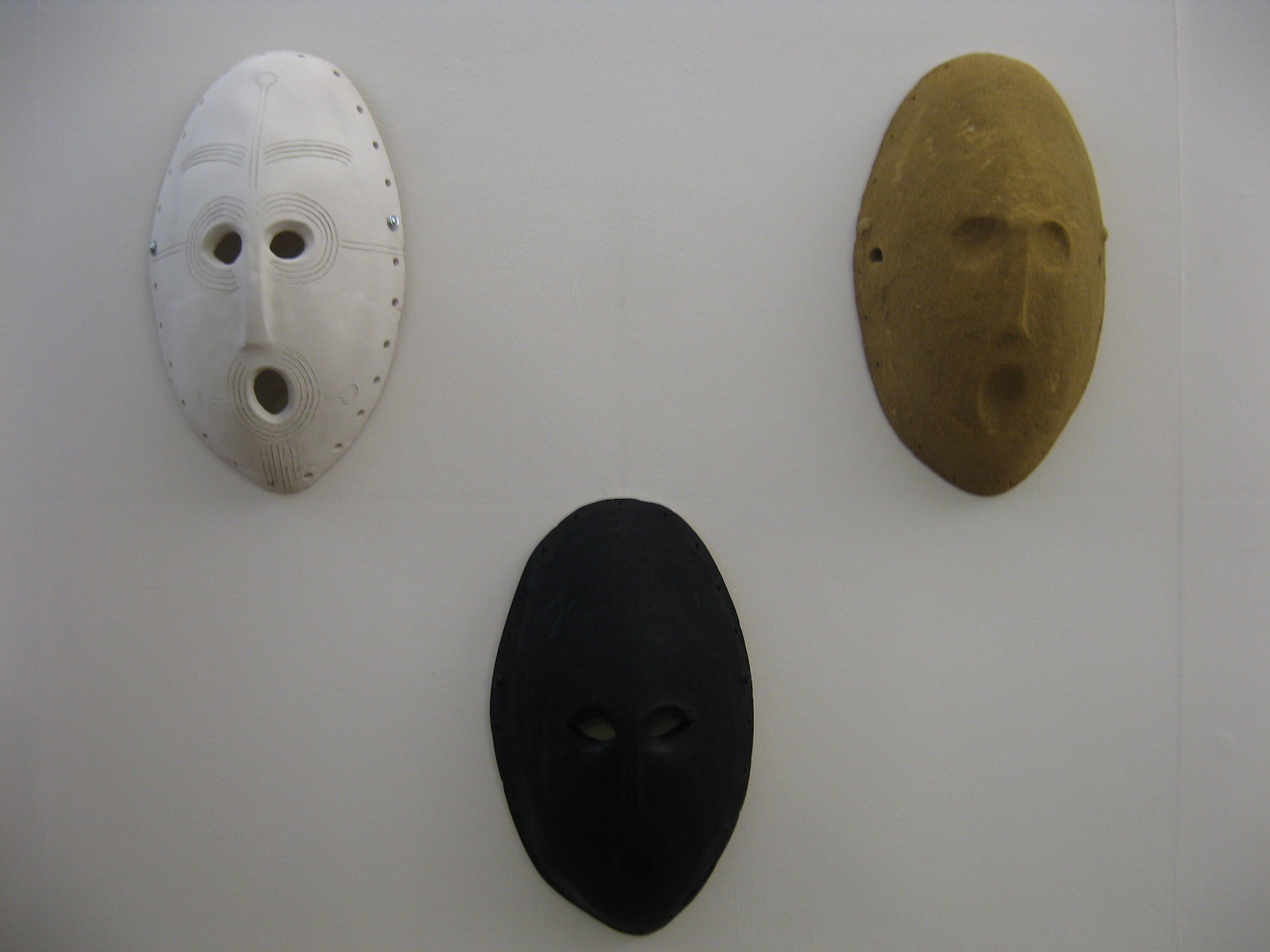The photograph showcases a collection of three distinct African-style tribal masks mounted on an off-white wall, organized in a triangular formation. The upper row features two masks while the lower row displays one centered beneath them. The top-left mask, crafted from pottery, is white in color with intricate details. Its design includes horizontally-elongated eye openings bordered by circular engravings, a rectangular nose, and an oval mouth encircled by etched lines that suggest a beard. Curved lines are etched above the eyes to resemble eyebrows, and small holes punctuate the mask's perimeter, likely for attachment. To its right, the second mask shares a similar size and shape but is hued in a dark clay brown. This mask is more plain, with defined indentations for the eyes and nose but without open eye holes, and a simple mouth feature. The single mask in the bottom row is entirely black and minimalist, its surface interrupted only by small eye openings, devoid of other distinguishing features.